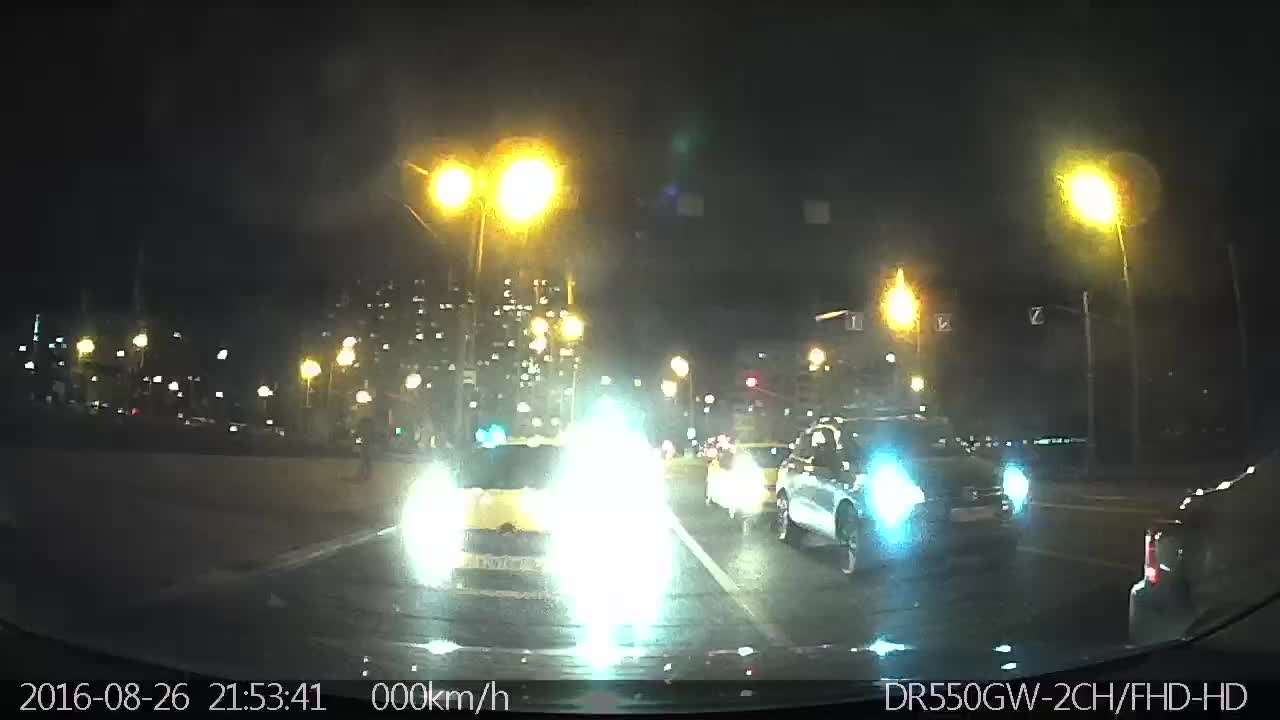An atmospheric nighttime street scene under a pitch-black sky, illuminated by the glow of city lights from tall buildings in the background. Streetlights cast a warm, diffused light over the road, revealing cars positioned in the foreground with their headlights on, facing towards the viewer. On the lower right corner, the partial rear end of a car is visible, followed by two additional vehicles with their lights on. In the left lane, there is a distinctive yellow car, also lit up. White lines clearly demarcate the lanes on the street. Under a streetlight positioned to the left, the silhouette of a person can be discerned against the darkness. Overlaying this urban tableau, white text at the bottom of the image reads: "2016-08-26, 21:53:41, 0-0-0 KM/H" to the left, and on the right, "DR-550GW-2CH/FHD/HD."